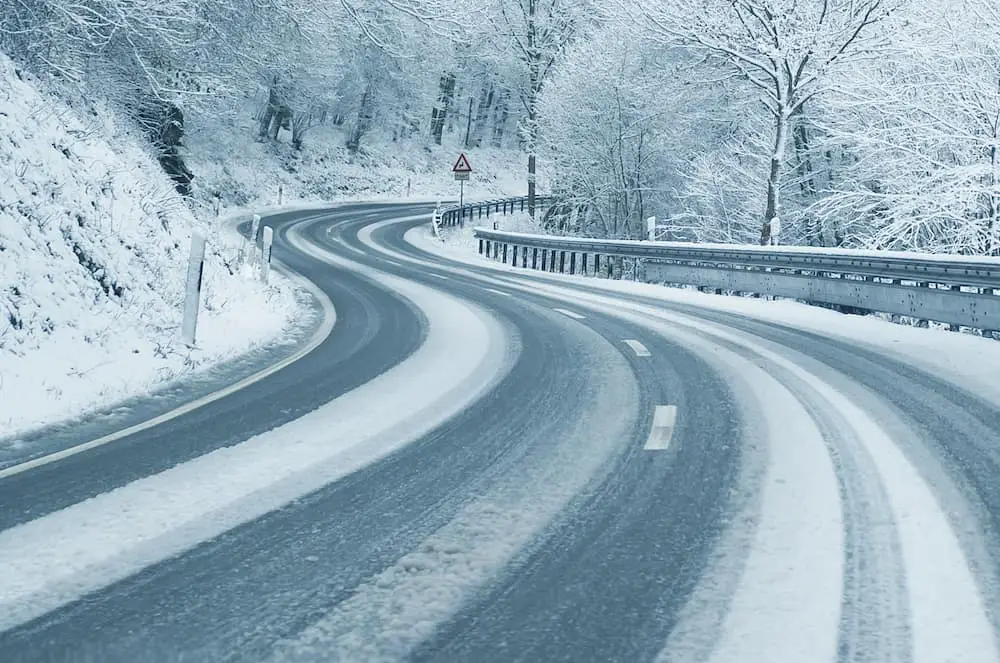This black-and-white professional photograph captures a picturesque winter scene along a winding, snow-covered mountain road. The road, which is in a rural area and appears well-traveled but still layered with snow, snakes through a dense forest of bare trees heavily blanketed in snow. It features noticeable tire tracks indicating prior traffic. To the right, a guardrail follows the bends of the road, showing signs of possible previous accidents with an open section suggesting a damaged area. Reflective poles are positioned along the left-hand side, enhancing the visibility of the road’s edges. A cautionary traffic sign is visible past one of the curves, likely warning drivers about the winding nature of the road ahead. The combination of bare, snow-laden branches and the twisting pathway creates a serene yet slightly treacherous atmosphere, evoking the essence of a winter wonderland.